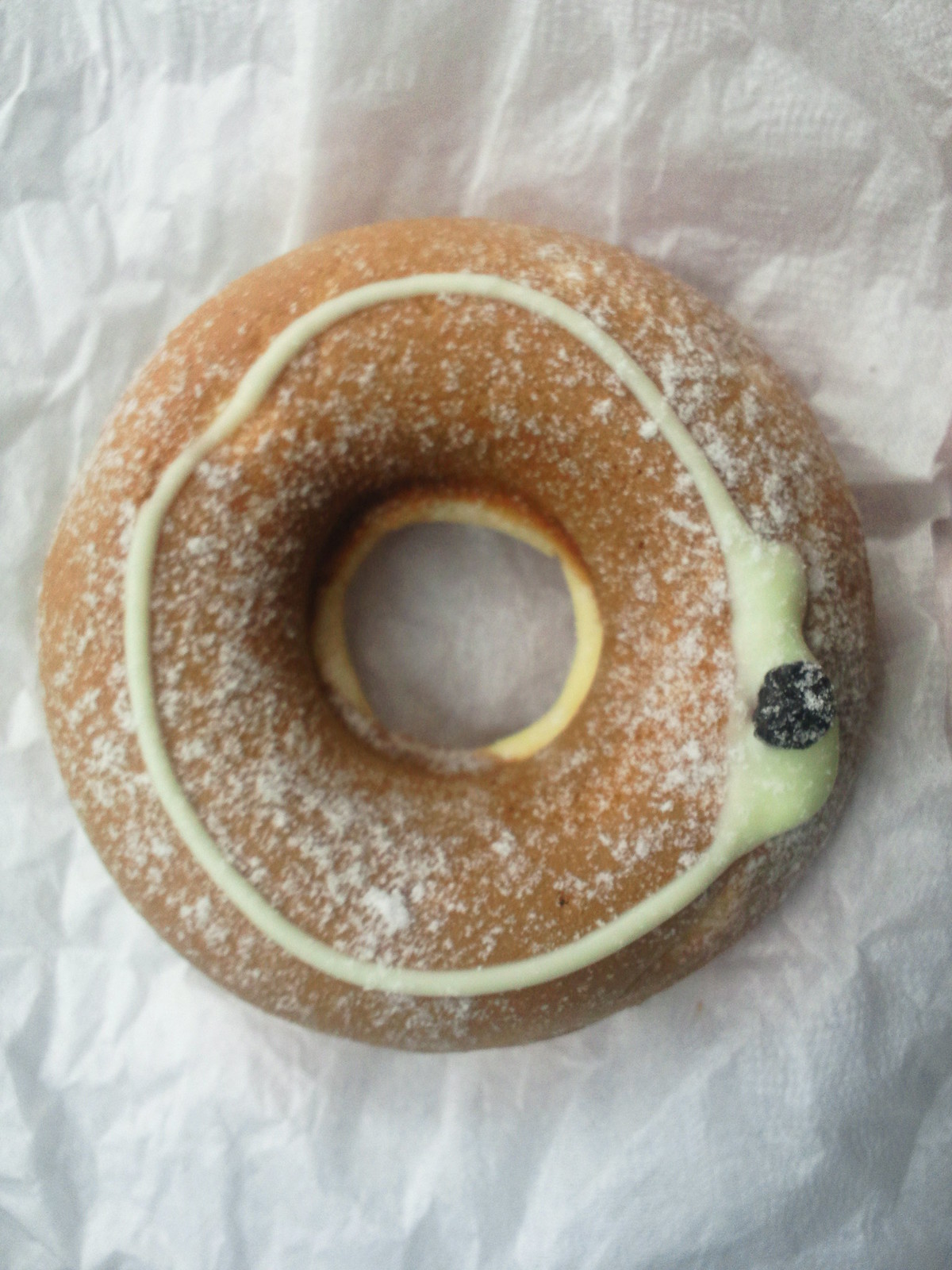This photorealistic image depicts a close-up, top-down view of a light brown donut centered in the frame, resting on a crinkled white paper towel. The donut is generously sprinkled with sugar, which accentuates its texture without completely masking its brown color. A distinct white icing encircles the donut, cutting through its middle circumference. On the right side, this icing thickens into a rounded area, where a small, dark shape, potentially a raisin or chocolate chip, is embedded and partially coated with sugar. The crisp white background and the crinkled paper towel contribute to the simplicity, keeping the focus on the clearly detailed donut.